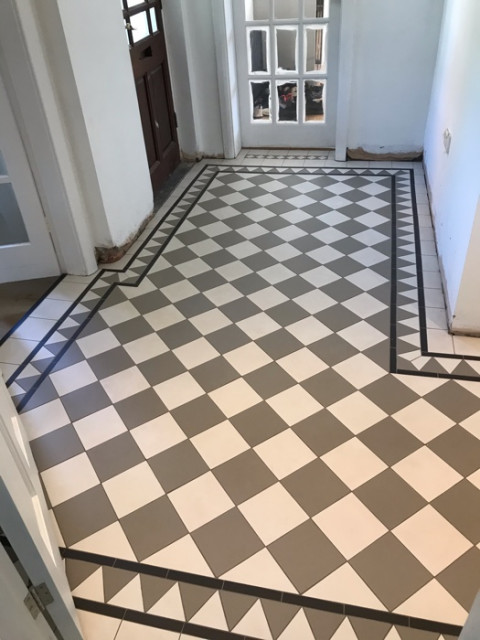The image depicts an entrance hall, likely to a home or possibly an apartment building, with no people or text present. Dominating the scene is a distinctive gray and white checkered floor pattern, arranged in a checkerboard design with squares or diamonds. This pattern is outlined with double gray lines and bordered by alternating gray and white triangles, separated by thin black tiles. 

Visible are three distinct doors: a set of double doors on the left with white trim, paralleled by a darker brown door without visible trim, potentially the main entrance. In the background is another door featuring at least nine window panels, allowing some transparency. All of these doors are in contrast with the stark white walls. Additionally, there seems to be an electrical outlet on the upper left wall. 

The floor extends beyond the picture's frame, suggesting additional doorways or a further hallway unseen in the image, while a hinge suggests a nearby door on the lower left side. The overall color scheme includes shades of gray, white, and black, adding to the sophisticated, somewhat stark ambiance of the entryway.